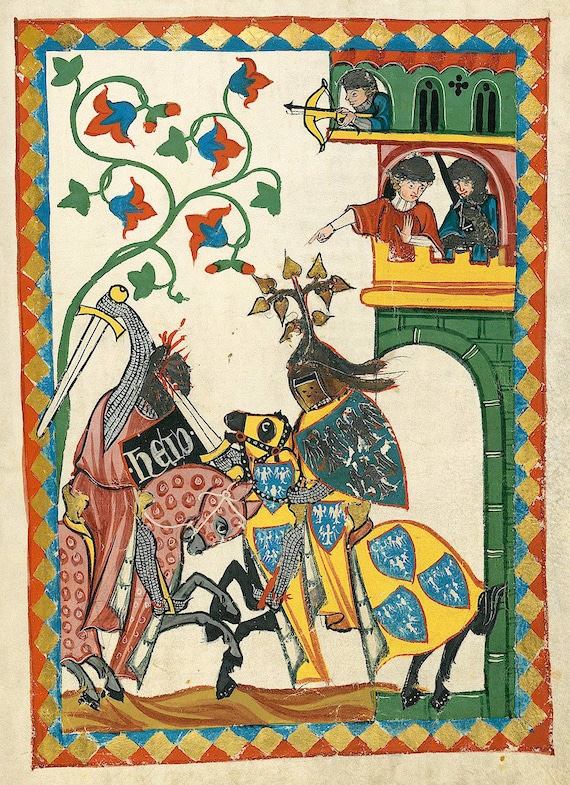The image is a detailed tapestry with a complex scene bordered by a pattern of red, blue, and orange diamonds. The central background is white, giving prominence to the depicted events. At the top of the tower, constructed of green bricks, stands a man in blue aiming a golden bow and arrow, his stance watchful. Below him, in a large red arched window, two men observe the action below. One wears a red and white top with a black hat, the other a blue top with a black hat. 

The first floor is also green and features a dramatic joust between two knights on horseback. The knight on the left rides a red horse and dons red and black armor, wielding a white and gold sword. He faces a knight on a black horse draped in yellow and blue fabric. The black horse has blue shields as part of its covering. The knight on the right is armored in a blue and yellow ensemble, adorned with an intricate helmet featuring arrow-shaped metal spikes. His sword, pointing downward, pierces through his adversary’s helmet, vividly depicted with red blood spurting out.

The scene is rich with medieval details, including a vine of red flowers and blue shields enhancing the medieval ambiance. The ground beneath the horses is uneven, accentuating the chaotic nature of the battle. The border frames the tapestry with a blue line, overlaid with a repeating pattern of gold diamonds, adding to the ornate tapestry's grandeur.